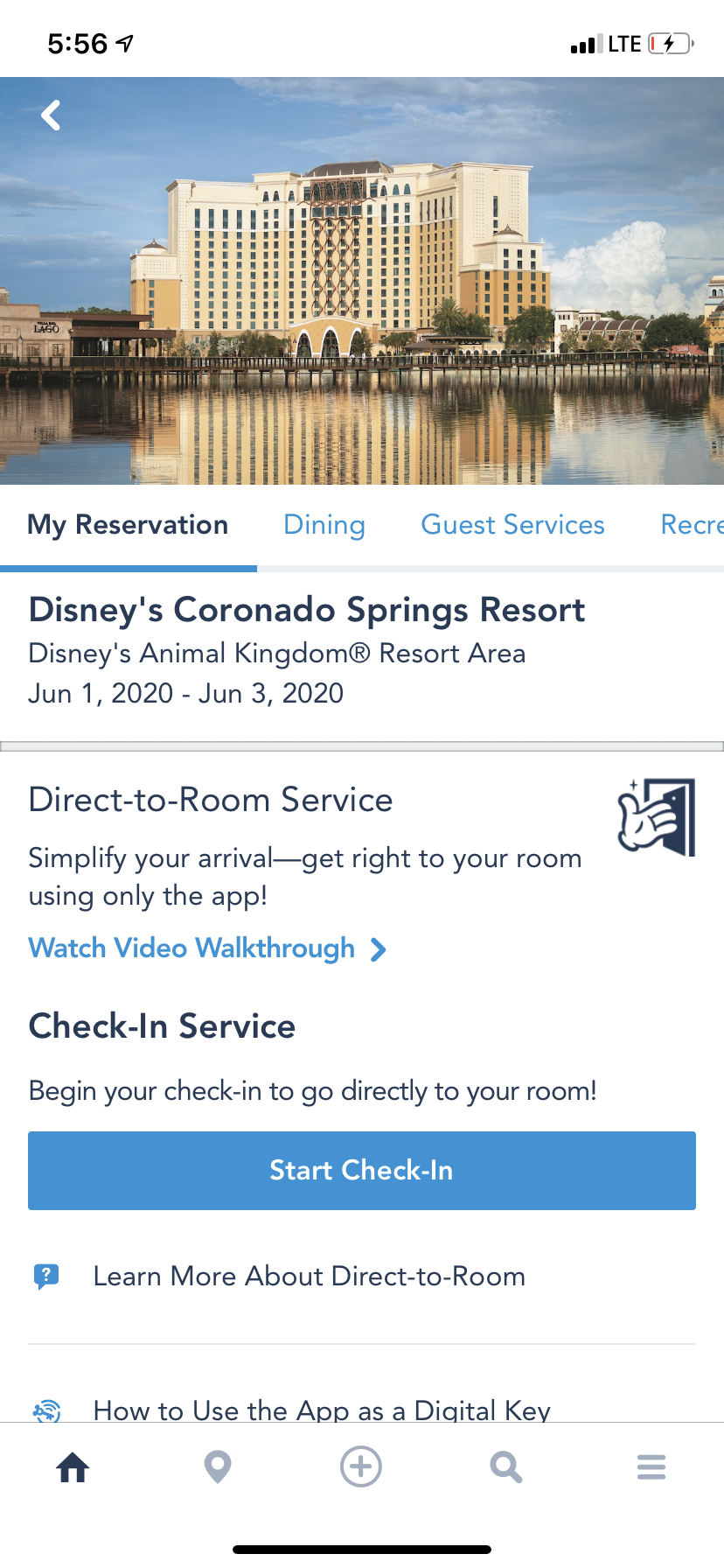Displayed on a mobile device, the website showcases essential details prominently. At the top-left corner, the number "556" is visible. On the right, icons indicate battery life and mobile signal strength.

The primary image at the top features a serene scene of a hotel or condominium complex with a beige and darker beige facade, set against a backdrop of a bright blue sky with scattered clouds. A vast body of water in the foreground reflects the building, adding to the picturesque quality of the photograph.

Beneath the image, the text "My Reservation" appears in black with a blue underline. Following this, options like "Dining," "Guest Services," and another partially visible category are listed in blue text.

The main heading, "Disney's Coronado Springs Resort," is written in bold black text, with "Disney's Animal Kingdom Resort Area" in smaller bold text below it. The dates "June 1, 2020 to June 3, 2020" follow, leading to a thin light gray bar spanning the screen.

Below the bar, a section titled "Direct-to-Room Service" encourages simplifying arrival with a description: "Get right to your room using only the app." An illustration of a gloved hand, reminiscent of Mickey Mouse, is shown pointing at an open doorway. The text "Watch Video Walkthrough" appears below in blue.

Further down, the "Check-In Service" title is in bold black text, prompting users to "Begin your check-in" and "Go directly to your room."

This detailed layout aims to provide a comprehensive and user-friendly overview for guests preparing for their stay at Disney’s Coronado Springs Resort.